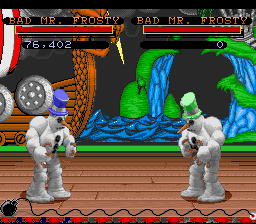In this still image from a video game, two snowmen characters are poised for battle, standing face to face on a platform made of wooden planks. Both snowmen boast exaggerated, circular, ball-shaped muscles on their arms, signifying their readiness for combat. One snowman is adorned with a purple top hat, while the other sports a green top hat. Each snowman features a prominent, long carrot nose. In the background, a majestic Viking ship sails, and a mysterious creature emerges from the water, adding an element of adventure to the scene. At the top of the screen, the text "Bad Mr. Frosty" is displayed along with two scores: 76,402 for one Bad Mr. Frosty character and zero for the other, indicating their ongoing battle within the game.